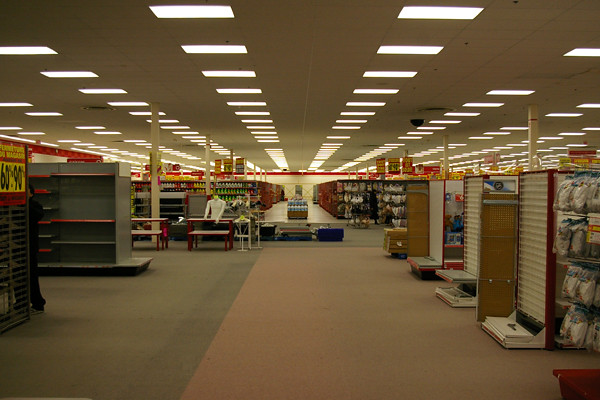This detailed picture was taken indoors at a department store, capturing a scene devoid of people. The central aisle, paved with reddish colored tiles, extends through the store, bordered by rows of empty shelves on the left and waiting-to-be stocked shelves on the right. The shelving units on the left are grey, while those on the right are a cream color. The ceiling is supported by thin cylindrical columns and is fitted with rectangular fluorescent lights. A striking red railing runs across the middle of the picture, adorned with various clipped signs advertising sales, including a prominent banner in red, yellow, and black, indicating discounts of 60 to 90% off. Just off-center, there stands a white, undressed mannequin next to a brown desk. Additionally, there's a pallet holding bottled water and several packages of white socks hanging in rows of four on the right. The floor area where these amenities are located is covered in gray carpeting.